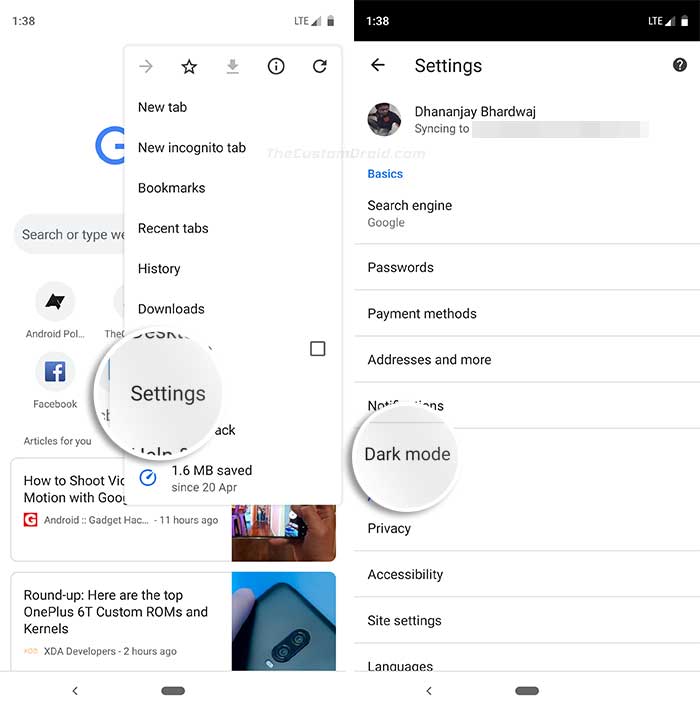The image displays multiple screenshots taken from a cell phone, showcasing various settings and options available within the device's interface. The primary focus of the image is on a specific settings page, which highlights the 'Dark Mode' option encircled for emphasis. This highlighted area is meant to guide users in enabling Dark Mode on their device. The background of these screenshots is predominantly white, with black text, except for hyperlinks, which are in blue.

Additionally, there is a circular magnification around the word 'Settings,' designed to help users easily locate this option on their device. This could be particularly useful for instructional purposes, as it visually guides users through the steps necessary to access settings and enable features like Dark Mode.

In the background, part of a Google search query is visible, indicating someone was searching for "round up here are the top one plus custom ROMs and kernels." Other visible elements within the settings interface include options such as 'New incognito tab,' 'Bookmarks,' 'Recent tabs,' 'Downloads,' 'History,' 'Search engine,' 'Passwords,' 'Payment methods,' 'Addresses and more,' 'Privacy,' 'Accessibility,' 'Site settings,' and 'Languages.' These additional options provide a comprehensive view of the various customizable settings available on the cell phone.